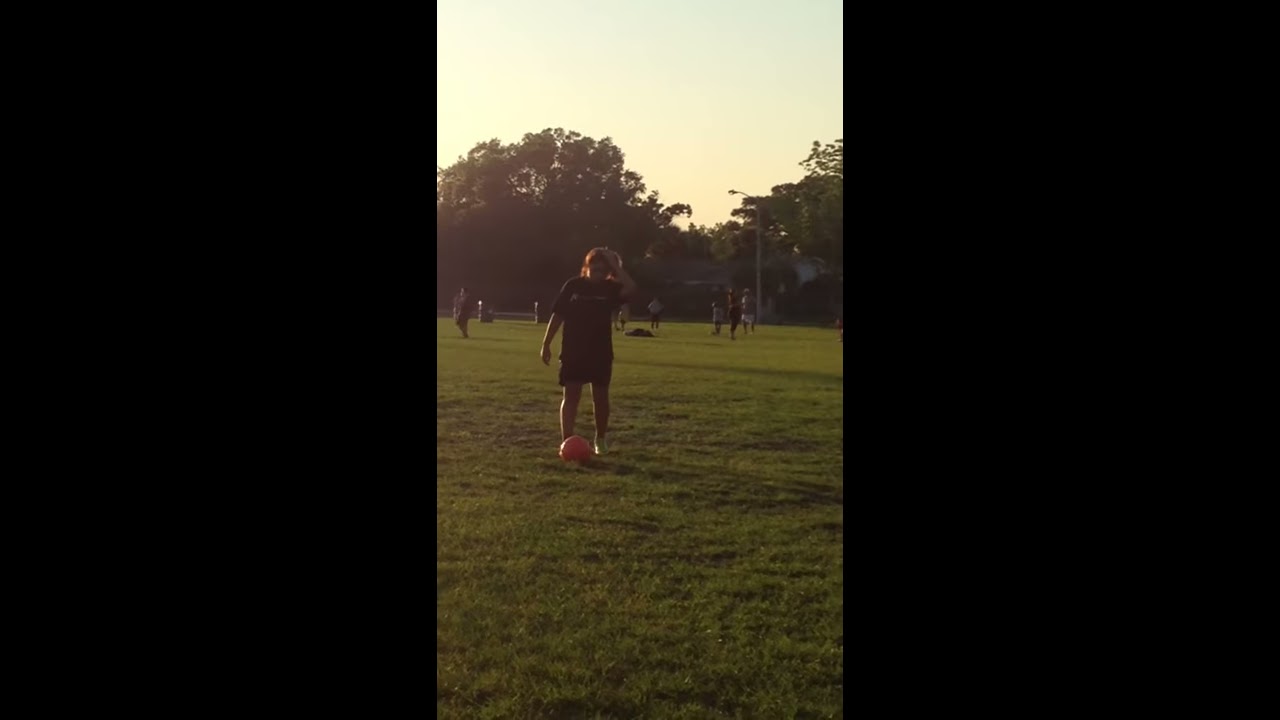The image captures a panoramic view of a sports field framed by solid black on the left and right thirds, bringing focused attention to the center. Set during a sunrise or sunset, the sky exhibits a beautiful orange and blue hue, with the sun shining low in the sky, casting long shadows across the field. The lush green grass of the field is scattered with a few distant figures suggesting either casual play or an ongoing game. In the foreground, a child, likely a young girl given her stature, stands prominently at the center. She's dressed in a black t-shirt and black shorts, her left hand resting on her head as she gazes down at an orange ball at her feet, poised possibly for a kick. To the right, a single lamppost stands tall among a backdrop of dense, leafy trees. The scene is imbued with a serene, almost ethereal quality, heightened by the sky's vibrant hues and the elongated shadows that hint at either early morning or late evening time.